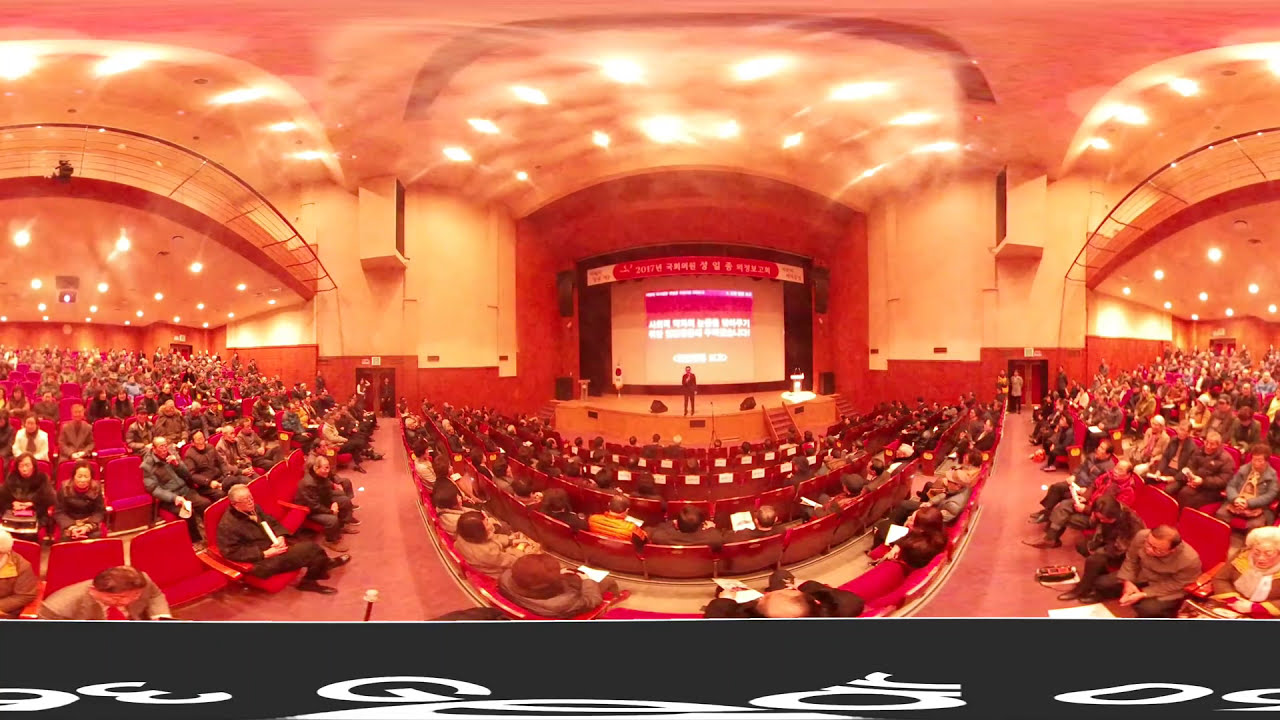The image features a fisheye lens perspective of a large auditorium or concert hall filled to capacity with mostly older attendees sitting in red seats. The seating is arranged in curved rows that encompass the central stage area, which is positioned against a backdrop of brown and beige walls. The room is brightly illuminated by numerous overhead lights, revealing a high ceiling. On the stage stands a solitary speaker holding a microphone, facing the audience. Behind the speaker, a large screen displays some indistinct text, which appears to be in an Asian language, along with possible graphic writing that reads "gear" or "gear 360." The immersive angle of the photograph accentuates the expansive and crowded nature of the venue.